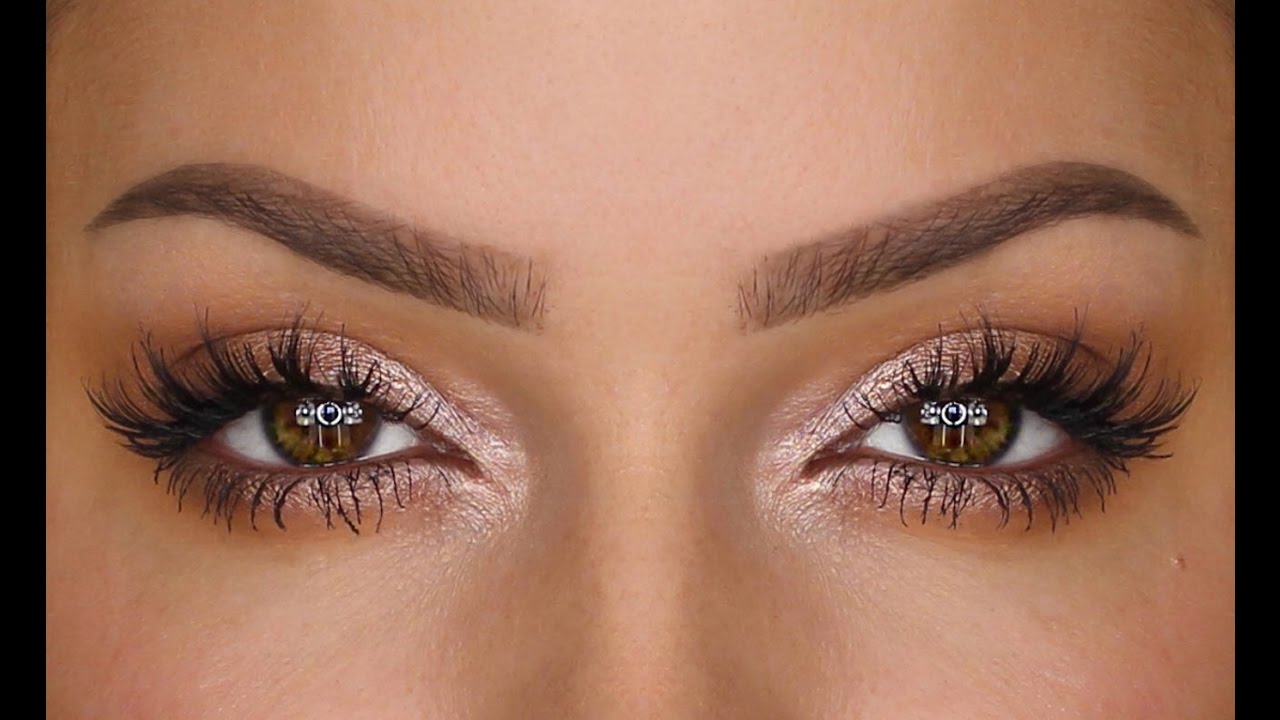The image is an extreme close-up of a feminine face, focusing solely on the eyes, eyebrows, the bridge of the nose, and part of the forehead. The individual's skin is tan, with a light brown hue. Her perfectly manicured eyebrows, enhanced with brown shading, appear almost painted on due to their precision. She is adorned with long, thick, and curled eyelashes that seem to be false, complemented by expertly applied, dramatic pink and brown sparkly eyeshadow. Her captivating brown eyes, which have reflections of white lights in them, are the focal point of the image, almost obscuring the dark pupils due to the intensity of the reflections. The overall makeup is meticulously done, creating a striking and polished appearance.